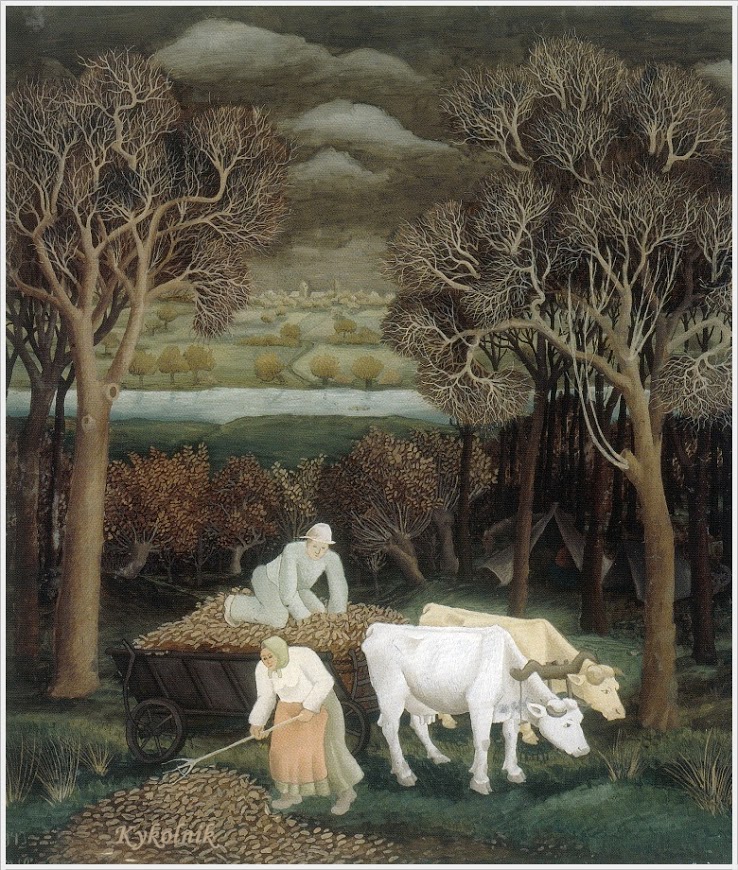In the detailed painting, a woman is seen raking leaves in the foreground while wearing a white shirt, a beige dress, a dark beige apron, and a tan handkerchief over her head. Nearby, a man dressed in a light-colored shirt, pants, and hat is on his hands and knees in a cart brimming with leaves. The cart is yoked to two oxen, one white and one tan, standing side-by-side. Their features, including the horns, ears, and eyes, are intricately detailed with smooth paint blending. The background reveals a landscape of barren trees in the foreground with more trees full of leaves further back, accompanied by rolling hills, a body of water, and tents visible to the right. Despite the detailed and bright characters, the overall tone of the painting is dominated by beige and gray hues, with dark, cloudy skies creating a somber atmosphere. The painting is signed "Kaikoulnik" and showcases a harmonious blend of light and dark elements, intricate tree branches, and a serene yet melancholic countryside scene.